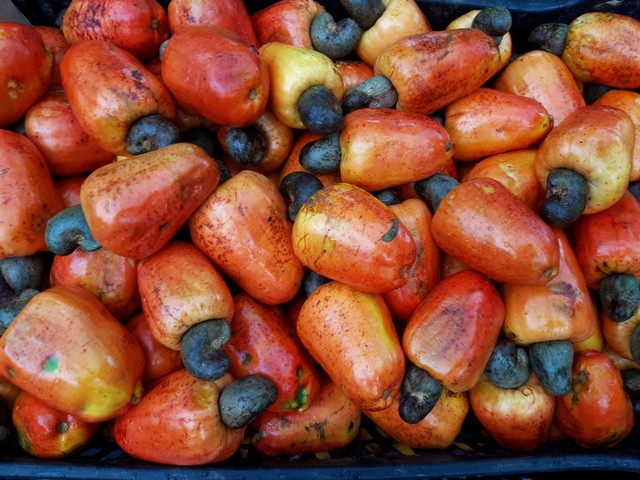The image features a close-up aerial view of a pile of red and yellow peppers, nestled in what appears to be a blue plastic basket. The peppers exhibit a gradient of warm colors, blending from red to orange to yellow, and each one has a distinct shape that is almost cylindrical with a slight taper, resembling a strawberry. Notably, every pepper is topped with a thick, curled brown stem, which ends in a round, brown bean-like shape, similar to a lima bean. Some of the peppers display imperfections such as scarring, blackened spots, or wrinkles, adding to the organic texture of the scene. The detailed arrangement within the basket, highlighted by visible slats at the edges, suggests a vibrant, yet natural collection of these intriguing fruits.